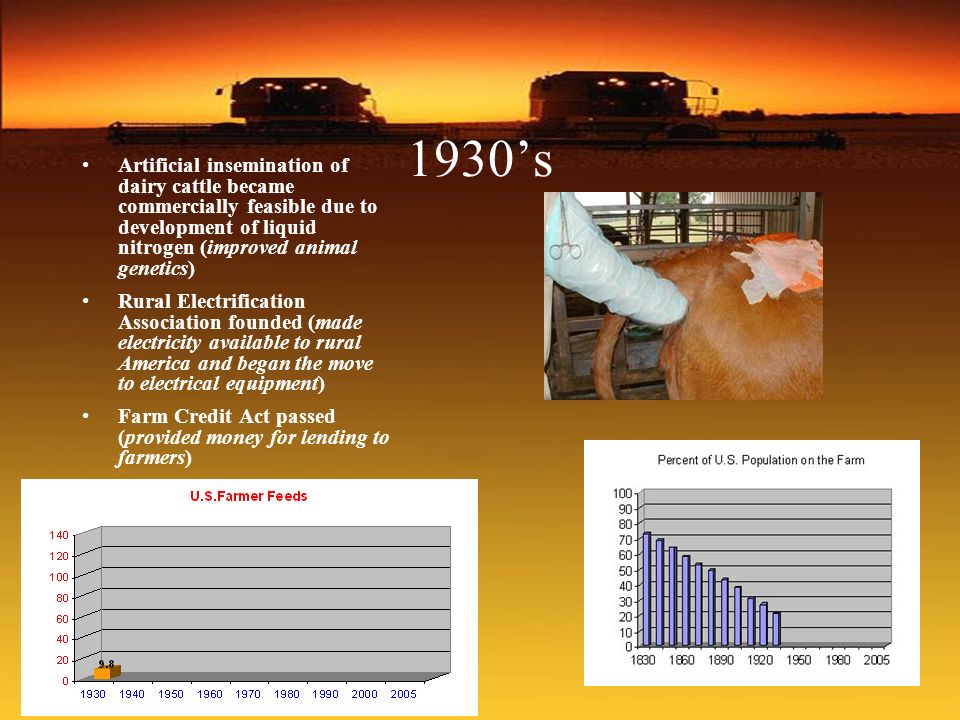This image is an informational graphic, resembling a research slide, with a collage of pictures and charts against a background of fields under an orange and yellow sky. In the upper portion of the image, two grain harvesting machines are shown operating in a farm field. Below this, a detailed section addresses the artificial insemination of dairy cattle, highlighting its commercial feasibility due to the development of liquid nitrogen and improved animal genetics in the 1930s. 
There is a notable picture to the right of center showing a veterinarian performing artificial insemination on a cow. White writing to the left details the prevalence of this practice since the 1930s and reasons for its adoption, such as the Rural Electrification Association's efforts, which brought electricity to rural America, enabling the move to electric equipment, and the Farm Credit Act, which provided financial support to farmers.

At the bottom of the image are two graphs: one showing the percentage of the U.S. population residing on farms from the 1830s to 2005, which indicates a significant decline over time, and another chart labeled "U.S. Farmer Feeds." This chart scales vertically from 0 to 140 in increments of 20, and the timeline at the bottom ranges from 1930 to 2005 in 10-year intervals.